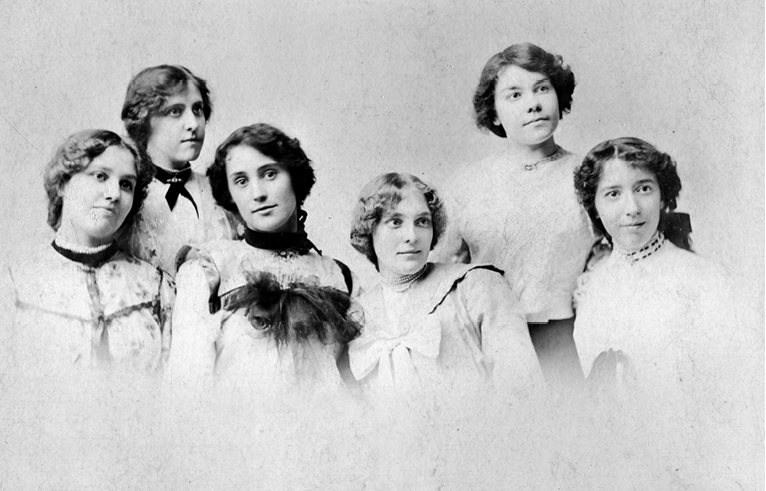This black-and-white photograph appears to be an old image, perhaps dating from the late 1800s to the early 1900s. The background is a mottled gray, and the picture captures six young girls, arranged in two rows with four seated in the front and two standing behind them. Their attire is characteristic of the era, featuring ornate and frilly blouses with high collars, some adorned with lace and bows. The girls have short, curled hair tucked beneath the nape of their necks, with variations in hair color ranging from brunette to possibly blonde. The photograph cuts off at the chest, leaving only their upper bodies visible. Most of the girls are gazing slightly to the right with soft, closed-mouth expressions, except for one positioned near the center who is looking directly at the camera. Despite the serious tones often captured in historical photos, these girls possess a gentle, relaxed demeanor.